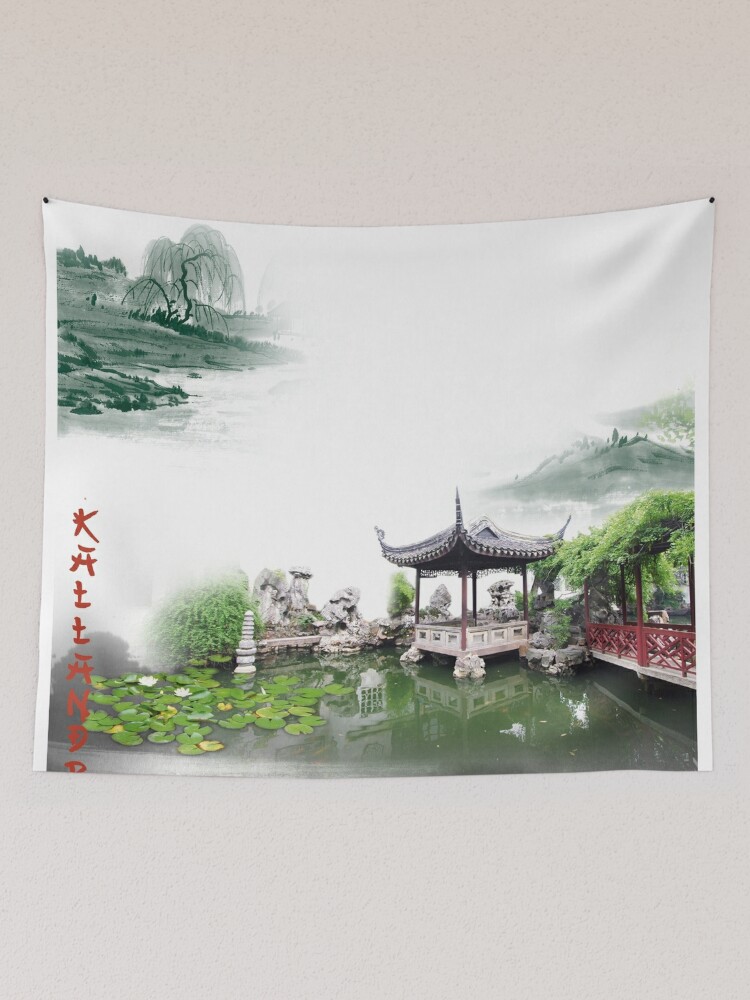The image is a detailed depiction on a white piece of textile material, possibly cotton or silk, measuring about 5 to 6 inches high by 4 inches wide. It is pinned to a light gray-pinkish wall using black pins in the upper left and right corners, creating a slight dip in the middle. The upper left corner of the textile features a dark green hillside with a weeping willow tree characterized by downward-hanging branches, all rendered in shades of green and gray. Prominent Japanese characters in red run vertically along the lower left-hand side of the fabric. The bottom part of the image showcases a serene pond adorned with lily pads and white lilies, extending towards the upper right. A stone pagoda with a pointed roof is situated on the water, accompanied by green plants and red fencing, surrounded by additional green hills in the background. The mix of painted and photographic elements enhances the intricate details and authenticity of the Japanese imagery.